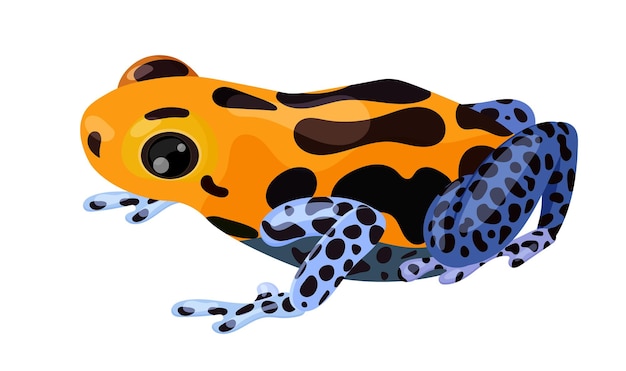The image depicts a colorful drawing of a small, frog-type creature set against a white background. The frog's main body is primarily orange, adorned with various black spots that range from round to irregular in shape. Its large, beady black eyes feature reflective dots, adding to its lifelike appearance. The frog's front legs are light blue with black spots and have webbed, three-pronged feet. Its hind legs are a darker blue, transitioning to a light lilac or purple at the feet, which also show black spotting. The creature appears to be poised on its front legs as if it is about to jump, showcasing a dynamic and lively stance.